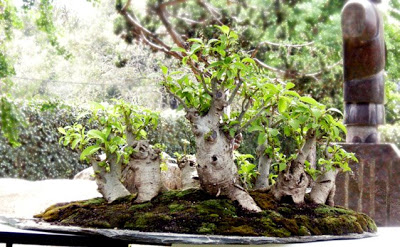A detailed and cohesive caption for the image:

The photo captures a tranquil garden scene bathed in sunlight, emphasizing a central circular area filled with both dirt and moss. Poking out from this earthy mix are several miniature trees, resembling young bonsai trees with white trunks and sparse leaves, indicating their youthful stages. The circular base hosting the bonsais appears to be positioned atop a table, contributing to its neatly contained look. In the background, there's an assortment of greenery, including taller trees and lush shrubbery, all contributing to the verdant atmosphere. Notably, behind the bonsai setup stands a wooden fence, and partially obscured by the foliage is a wooden statue with a strikingly phallic shape, adding an artistic element to the garden. The overall feel is one of serene nature and carefully curated plant life, typical of an ornate garden setting.